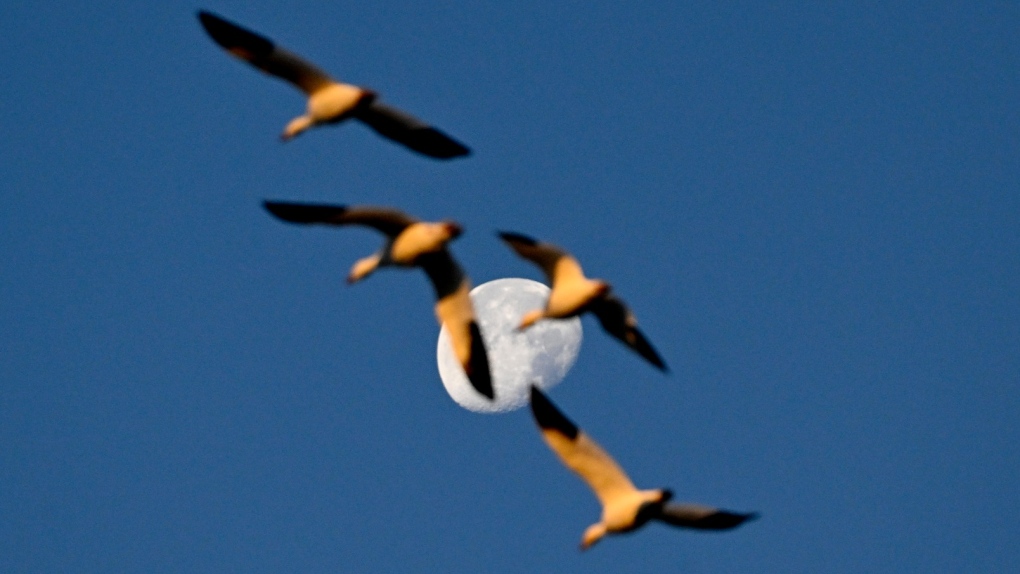The photograph captures a mesmerizing scene of four large birds flying across a dim, dark blue sky with an almost full moon centered prominently in the background. The birds, likely geese or similar species, are flying in formation from the upper left to the lower right, slightly staggered and with their wings extended. Although the birds in the foreground are out of focus, it is apparent that their wingtips are black, and their bodies and underwings exhibit a blend of yellowish-orange and pinkish-red hues, likely highlighted by the low sun. The moon, detailed with visible structures and craters, stands in sharp contrast to the blurred birds, creating a striking focal point in this horizontally landscape-oriented photograph. The sophisticated blend of colors on the birds and the clear celestial backdrop adds a captivating dynamic to the image.